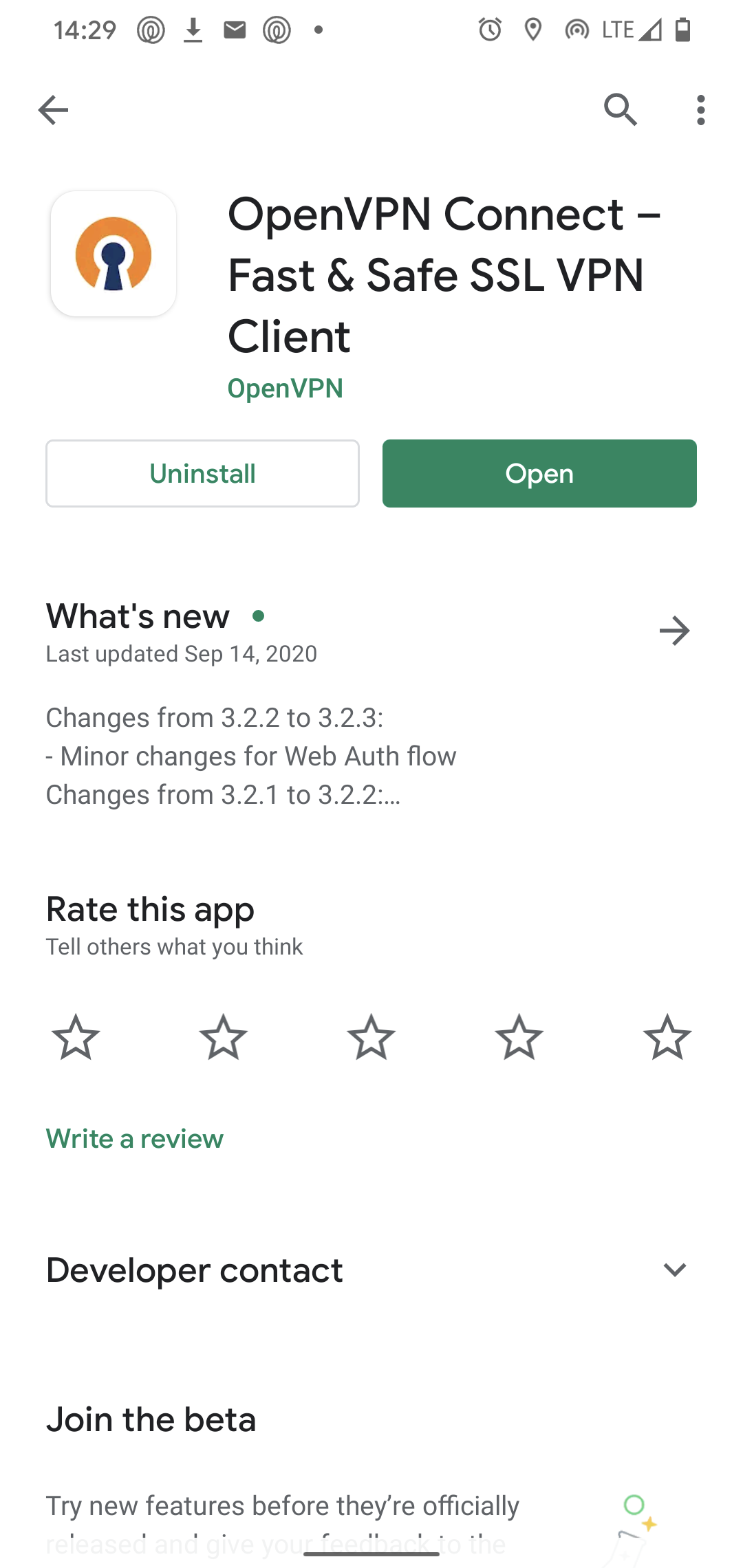The image being described is a smartphone screenshot showcasing the app interface for "OpenVPN Connect." The screenshot has a predominantly white background with black text. The dimensions suggest the image is significantly taller than it is wide.

In the top left corner, the time is displayed as "14:29" in black text, followed by about five notification icons. In the top right corner, several icons representing signal strength and battery life are visible. Below this, there is a navigation bar with a black left arrow on the left side, and a search icon along with three vertical dots on the right side.

Beneath the navigation bar, a logo representing the app is present. The logo features a keyhole within an orange semi-circle that is open at the bottom. To the right of the logo, the app name "OpenVPN Connect" is displayed in black text, with a subtitle in green text reading "Fast and safe SSL VPN client." Below this, a green text in bold reads "OpenVPN."

Two buttons are positioned below the app information. The left button is a white rectangle with green text that says "Uninstall," and the right button is a green rectangle with white text that says "Open."

Further down, there is a "What's new" section detailing recent updates over four lines of text. Following this is a "Rate this app" section featuring five outline stars for rating, with a green text link below it that states "Write a review." Lastly, there are links labeled "Developer Contact" and "Join the Beta" at the bottom.

The overall layout provides a clear and structured presentation of the app's essential functions and options.